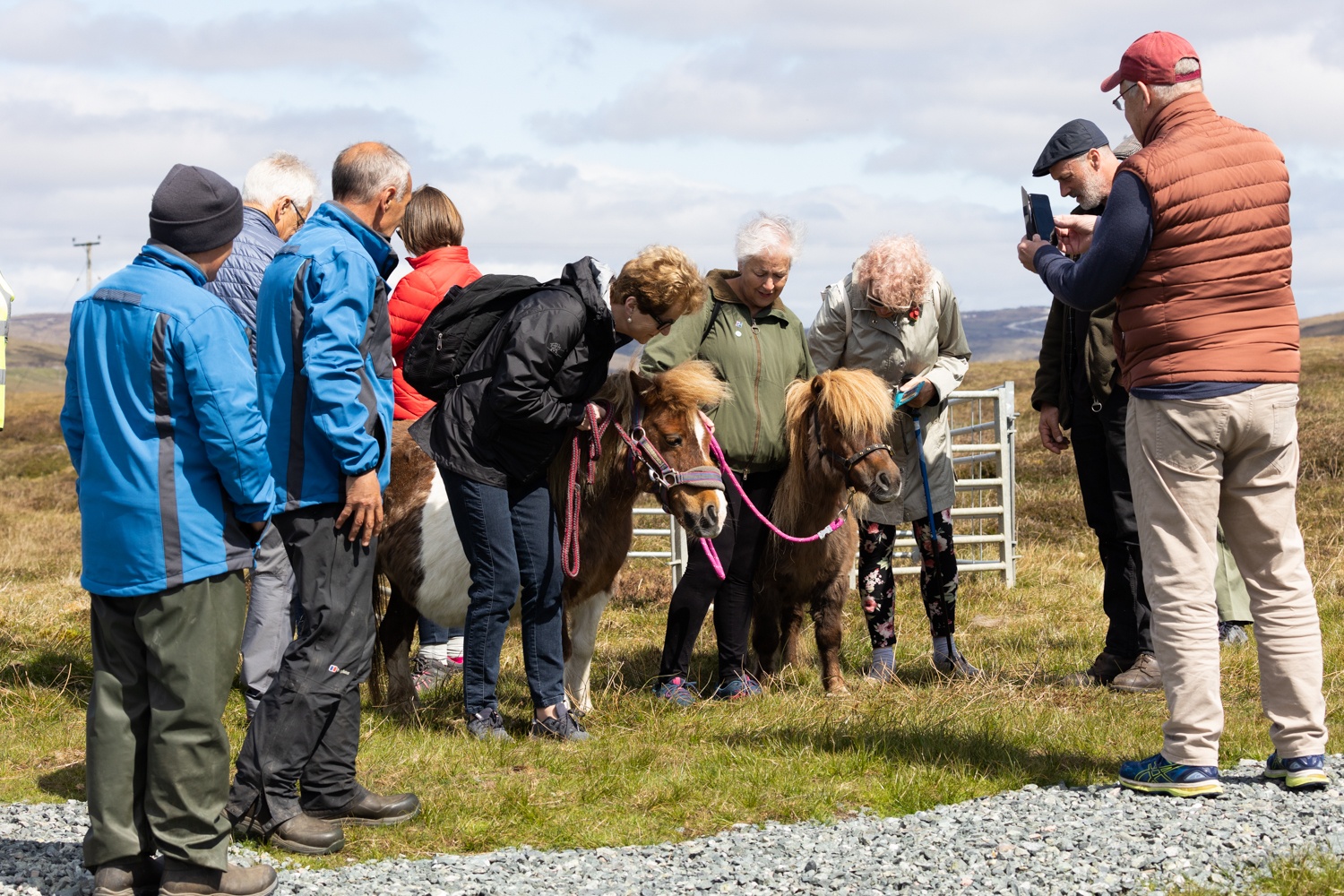The image captures a field scene where a diverse group of people is gathered around two small ponies. The setting is a green grass field dotted with patches of dry, brown grass and bordered by a white gated area and a gravelly, rock-strewn pathway. Above, the sky is a mix of blue and gray clouds, suggesting a chilly day as indicated by the attendees' warm attire—various jackets, vests, and hoodies.

At the center of attention are the two ponies: one is completely brown with a thick mane of hair on its head, while the other is a heavier-set pony with a mix of brown and white, also sporting blonde hair. The ponies are adorned with pink and purple halters, and some people appear to be holding their leashes.

In the group, notable figures include two men in blue jackets—one with gray slacks and the other with green—standing toward the left. Nearby, a woman in a black jacket and jeans with a backpack is bowing down, seemingly interacting closely with one pony. Another woman in a green hoodie and a second woman are on either side of the all-brown pony, likely petting it. Adding to the lively scene, some people in the background seem to be taking photographs, possibly capturing the interaction between the ponies and participants.